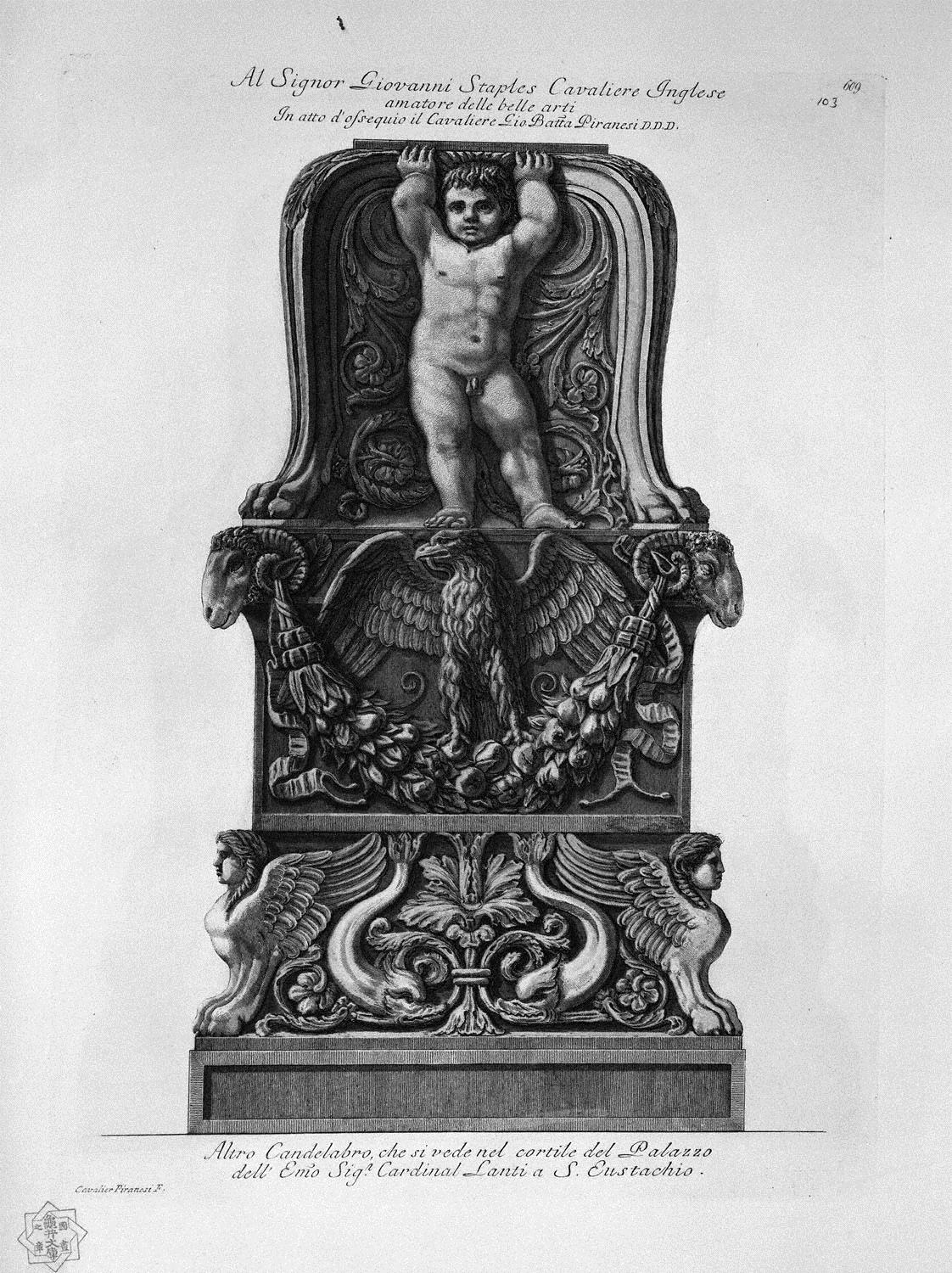This detailed black and white drawing appears to be a depiction of a heavily carved three-tiered candelabra or ornate pedestal, possibly from an illustrated book or catalog. The topmost level features a strong, portly cherub or baby, unclothed, holding up an intricate platform as if ready to support a candle. The middle section showcases a meticulously carved eagle with its wings fully spread, resting on a cascade of flowers that connect two detailed ram's heads on either side. The eagle's feathers are rendered in great detail, with each individual feather clearly visible. The bottom section displays two griffins with lion-like bodies, wings, and human female faces facing outward from each other, flanking an elaborate floral design that includes a fleur-de-lis motif. The entire structure is characterized by its extremely intricate and ornate carvings. Surrounding the image is text in Italian that reads "Al Signore Giovanni Staples Caravagli Inglese" and the number "102," suggesting this may be an item listed in an auction catalog or page 102 of a book. The piece appears to be made of wood, and the drawing captures the richness of the carvings in exquisite detail.